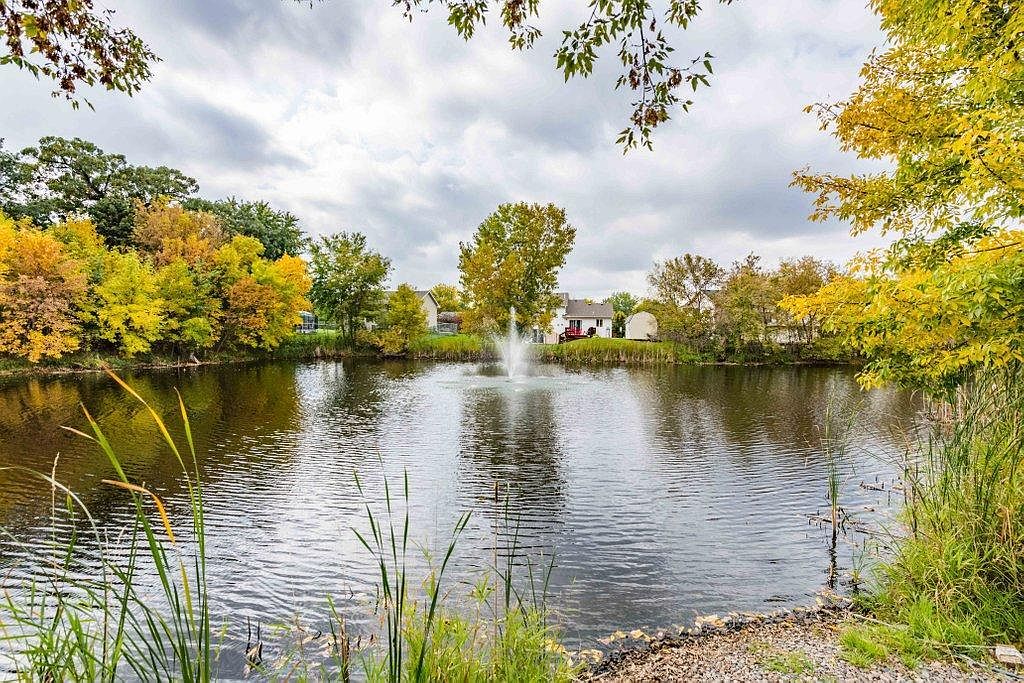This photograph depicts a picturesque, man-made pond with a central water spout fountain, spraying white water high into the air. The pond's surface, a light green hue, reflects the large, thick gray and dark gray clouds in the light blue sky above. The shoreline is adorned with small pebbles interspersed with water plants, including reeds and tall grasses, creating a lush natural border. Surrounding the pond are multiple trees in full autumn splendor, their leaves vibrant shades of yellow and orange. On the far side of the pond, several residential single-family homes, including a prominent multi-story white house, stand behind the trees, adding a touch of human presence to the serene landscape. The combination of the rippling water, colorful foliage, and homes in the background captures a tranquil, autumnal scene.